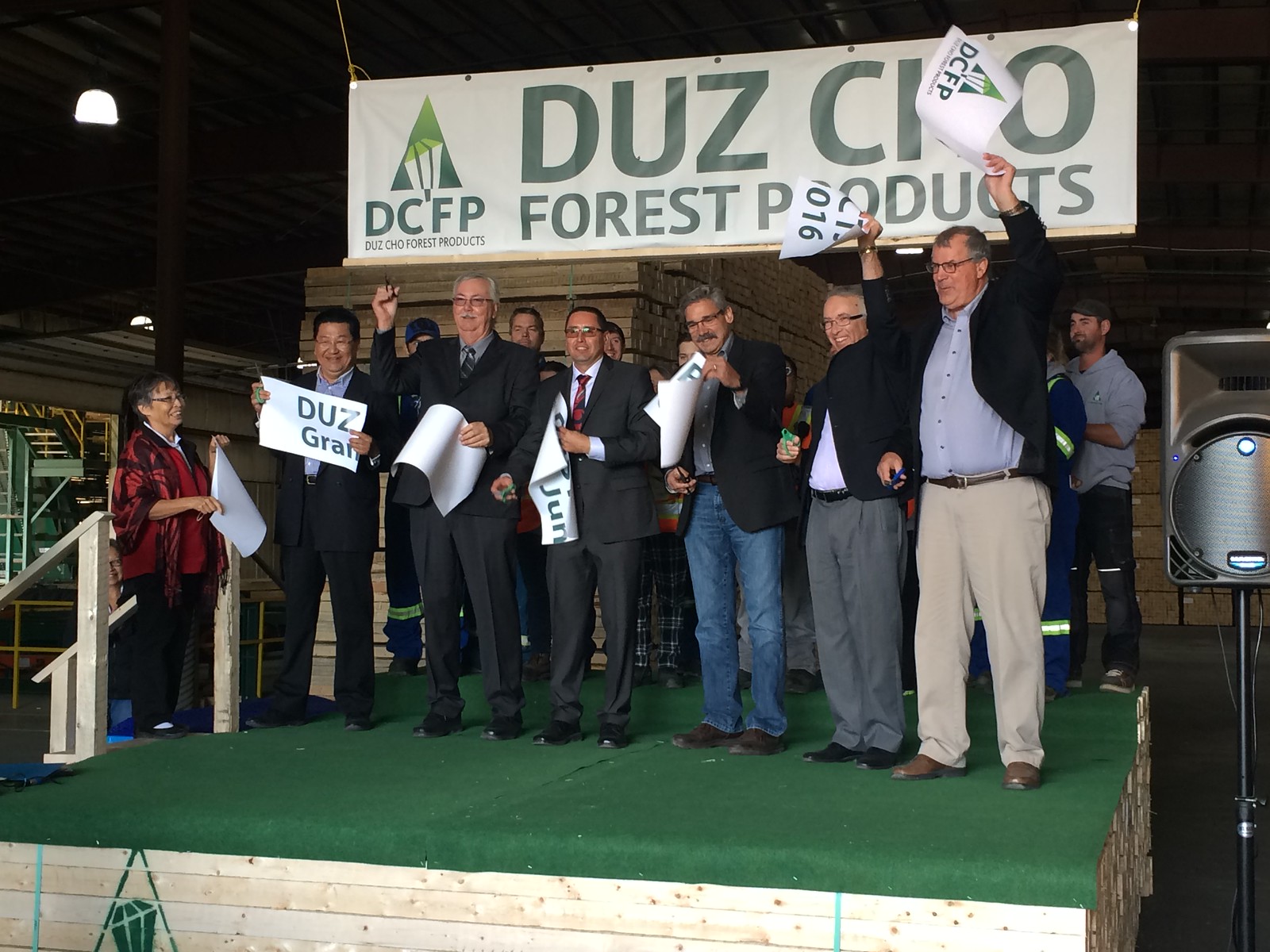The image captures a scene inside a warehouse where about a dozen men, dressed in suits or dark jackets, are standing on a makeshift raised platform made of pale wooden boards. The platform is partially covered with a green fabric, and a handrail constructed from the same boards is visible. One woman, dressed in red, is standing on a set of wooden stairs leading up to the platform. The men are holding white papers bearing the text "Dues Grant" and "DCFP" in green font, waving them in celebration. Hanging from the ceiling above is a large white banner that reads "Dues CIO Flores Products." In the background, the warehouse is filled with stacked wooden boards and boxes.